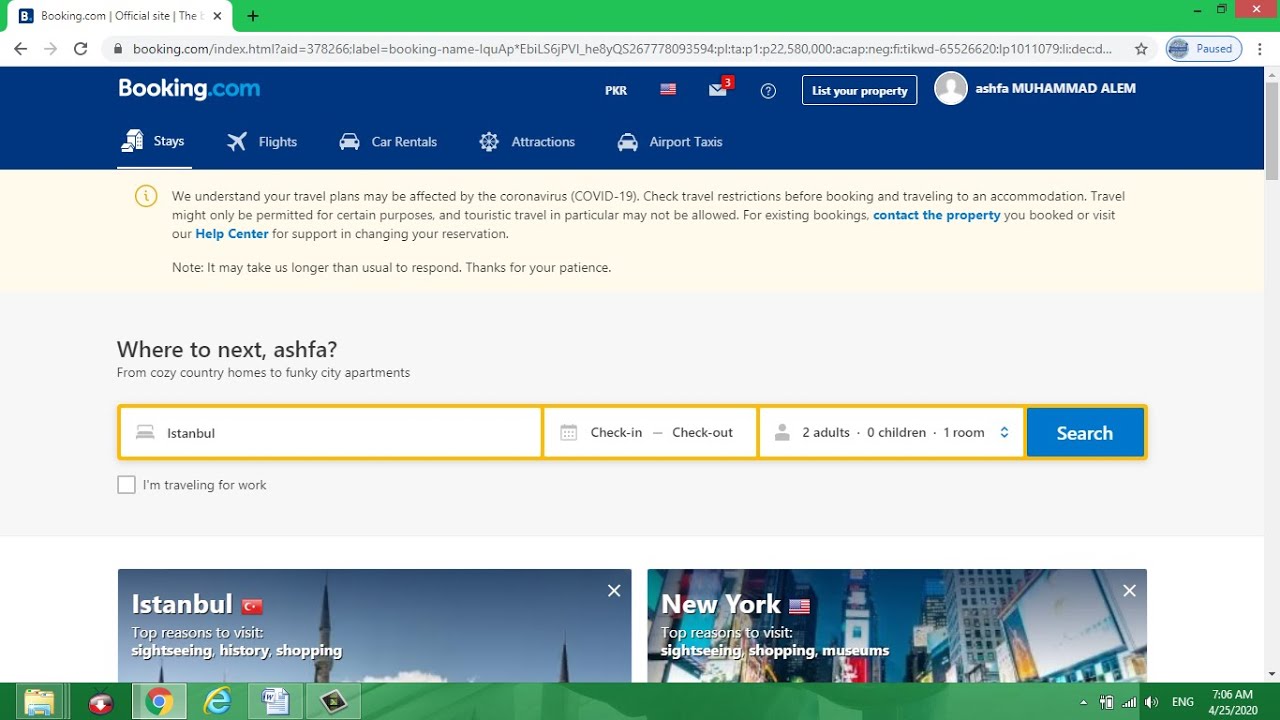The image depicts the homepage of Booking.com, a popular travel website. At the top, there's a navigation bar featuring different categories such as stays, flights, car rentals, attractions, and airport taxis. The navigation bar is set against a deep royal blue background, which transitions to navy blue, and is bordered by a slimmer, green rectangle on the top. The Booking.com logo is displayed prominently, with "Booking" in white and ".com" in a lighter blue color.

Beneath the navigation bar, there's an important message addressing the potential impact of the coronavirus on travel plans. Below this message, there's a prominent search section with the prompt "Where to next, ASHFA?" encouraging users to explore a variety of accommodations, from cozy country homes to funky city apartments. In this section, someone has entered "Istanbul" as their desired destination, and there are fields to input check-in and check-out dates, as well as the number of adults and children traveling. A search button is available to initiate the search for accommodations.

At the very bottom of the image, there are captivating photographs of two major cities: Istanbul and New York, enticing travelers with visual previews of these popular destinations.